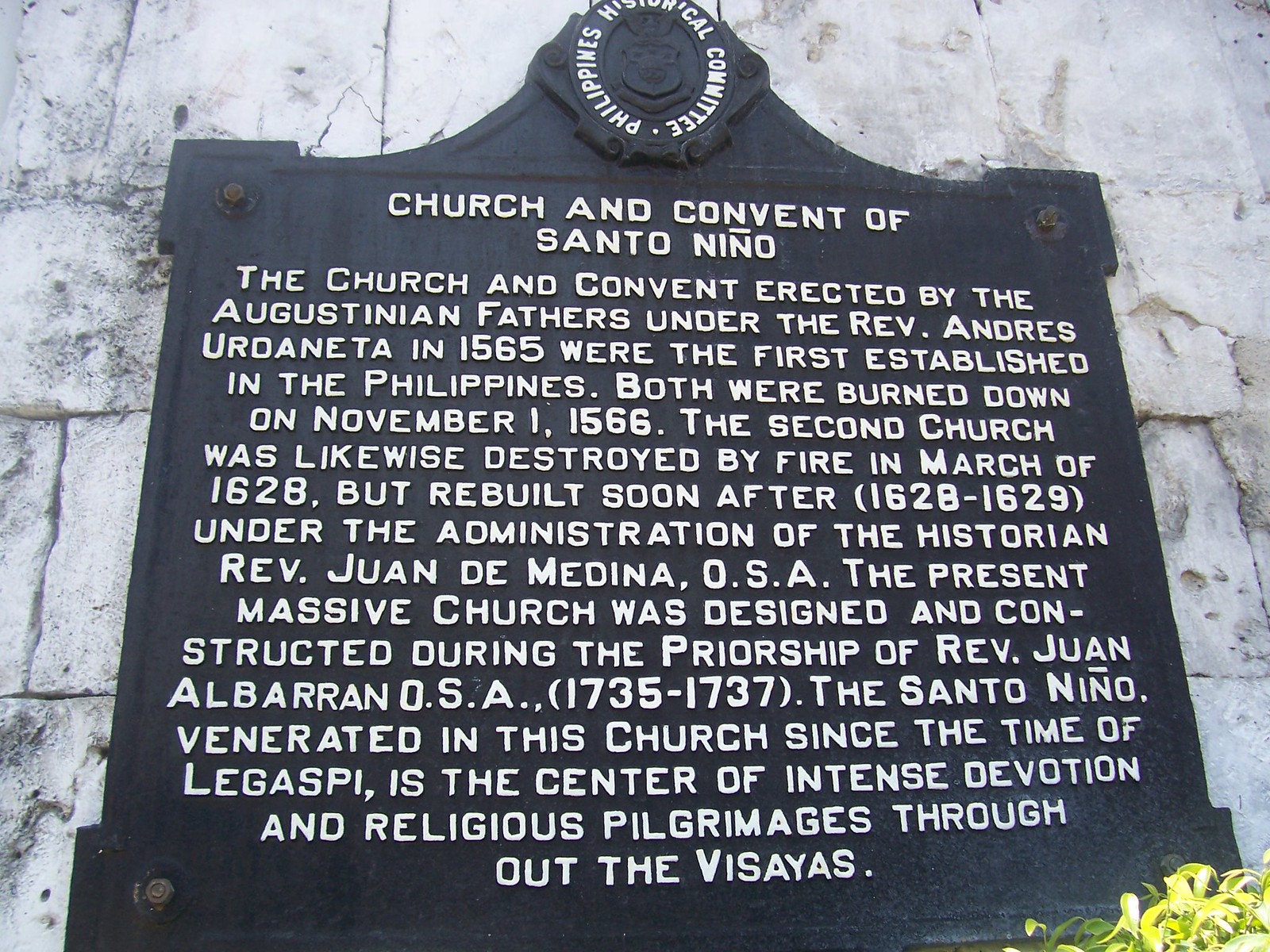This color photograph captures a detailed view of a historical black metal plaque mounted on a white stone wall, with a green plant visible in the lower right-hand corner. The plaque, which is affixed with metal fasteners, prominently features a raised badge with a crown at the top center, inscribed with "Philippines Historical Committee" in a circle. Below this emblem, the plaque states: "Church and Convent of Santo Niño." The inscription details that the Church and Convent were erected by Augustinian fathers under Reverend Andrés de Urdaneta in 1565, marking them as the first established in the Philippines. The text goes on to note that both structures were burned down on November 1, 1566. A second church, subsequently built, was also destroyed by fire in March of 1628 but was quickly rebuilt soon after.